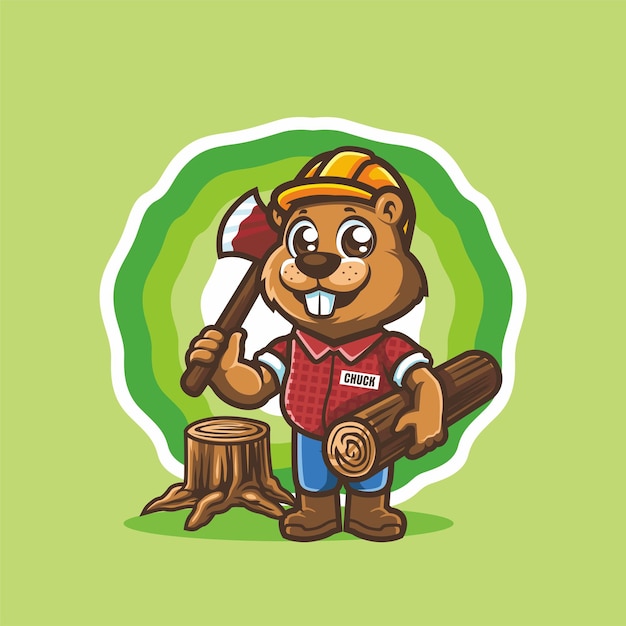This digital cartoon artwork features Chuck the Beaver set against a solid pea green background. Central to the composition is a multi-shaded green circle with alternating white, dark green, and light green bands, drawing attention to Chuck, who stands proudly in the middle. Chuck, a brown beaver with big buck teeth and expressive eyes, sports a yellow construction helmet and a red shirt with his name, "Chuck," emblazoned on it. He completes his outfit with blue denim jeans and brown shoes. In his left hand, he clutches a wooden log, while his right hand wields a red axe with a silver edge. To the left of Chuck, there's a tree stump with visible roots, adding a rugged, forestry vibe to the scene.